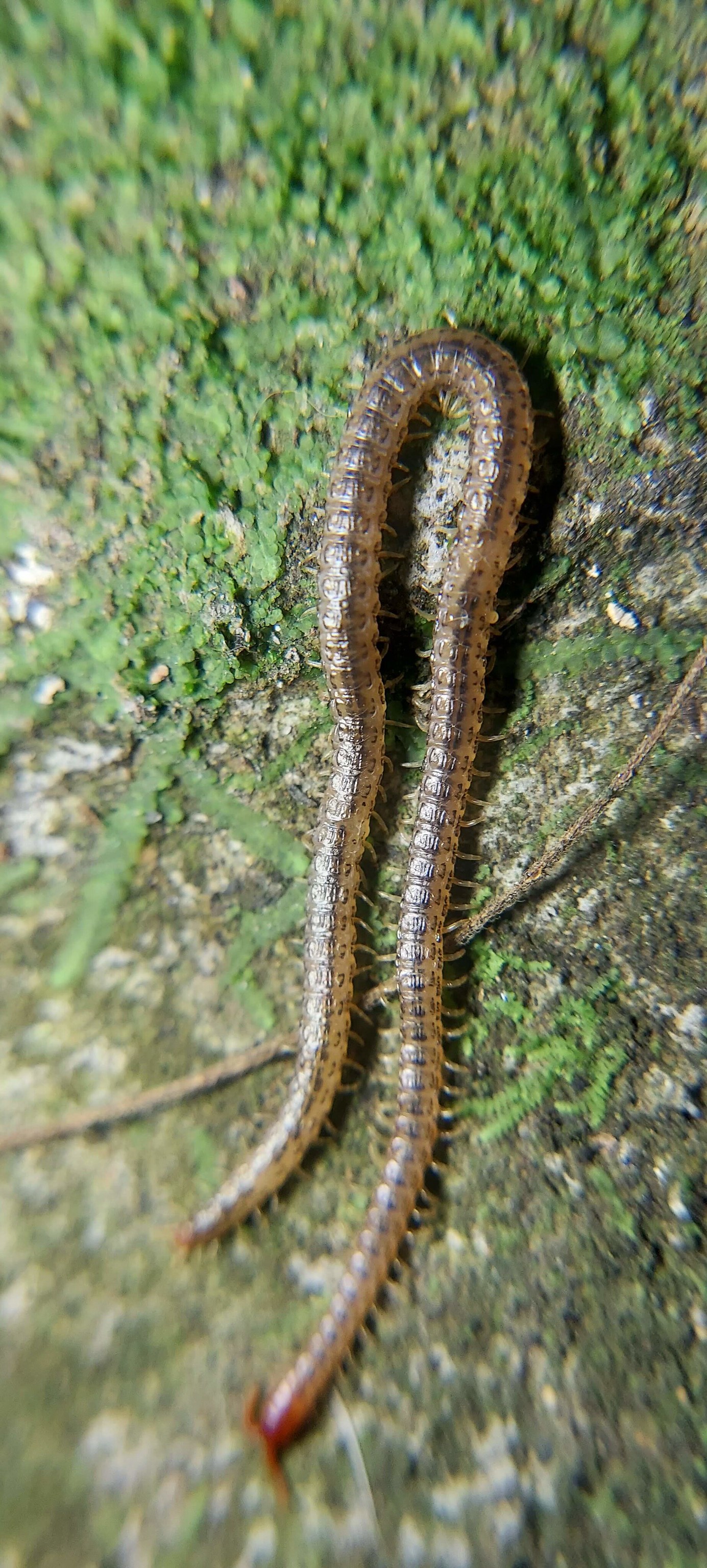The photograph captures a detailed close-up of a lengthy, many-legged insect, likely belonging to the centipede or millipede family. This worm-like creature is distinguished by its hundreds of slender legs extending from its beige and brown body. The insect, which features a notable red coloration at one end (likely its head), is arched in an upside-down U-shape. It rests on a moss-covered rocky surface, lending a vibrant green backdrop contrasting with the rock's gray and white hues. The image is vertically oriented, with a focused middle section highlighting the insect, while both the top and bottom portions appear blurred. A small brown stick is also visible across the middle of the frame, further adding to the intricate details of the rocky, mossy environment.